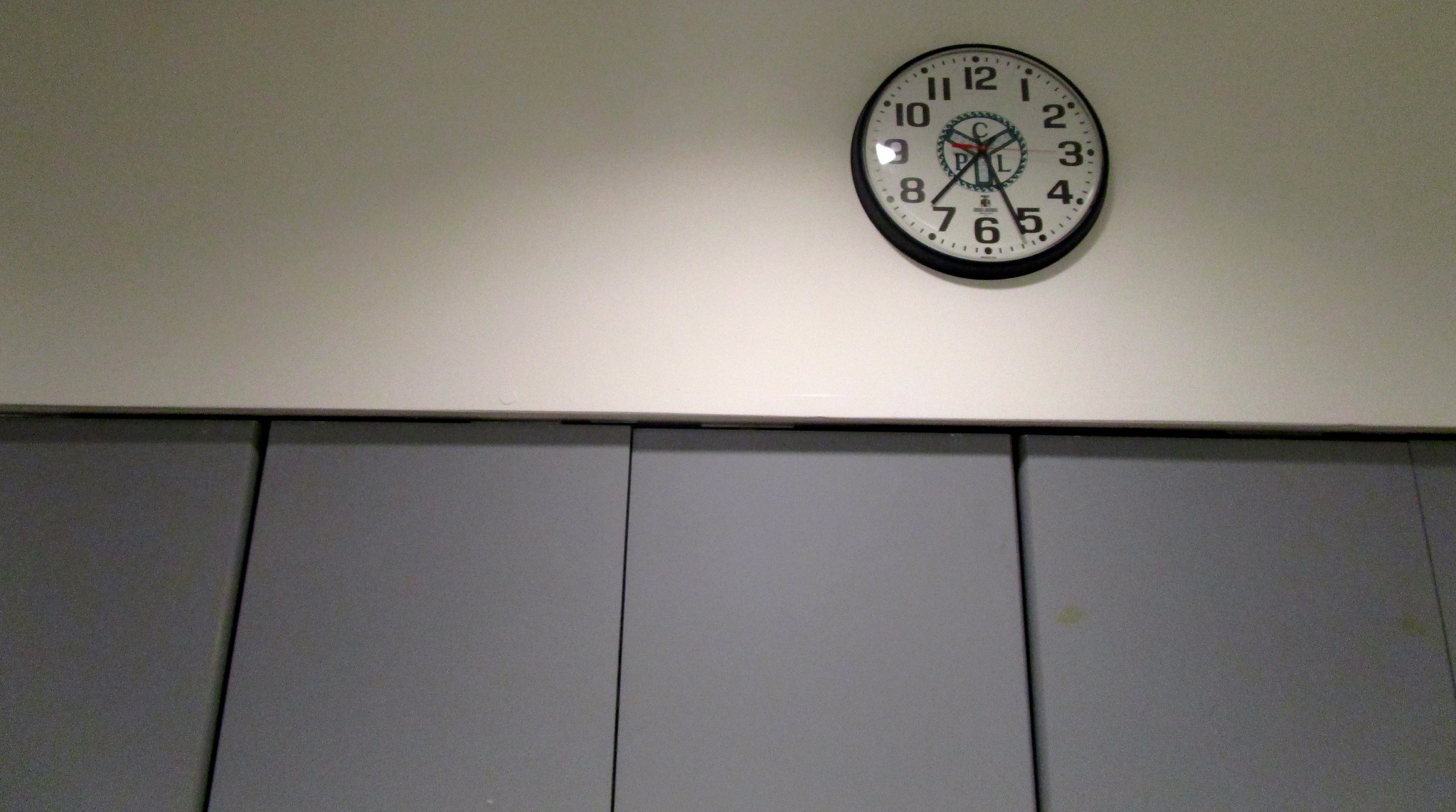The image shows a white wall adorned with five gray panels, likely used for soundproofing. The panels are partially visible, with the fifth panel barely making it into the frame on the right-hand side, and the first panel appearing halfway on the left. Above the panels, there is a classic, round school clock. The clock reads 7:36 and has the letters "CPL" prominently displayed in blue at its center.